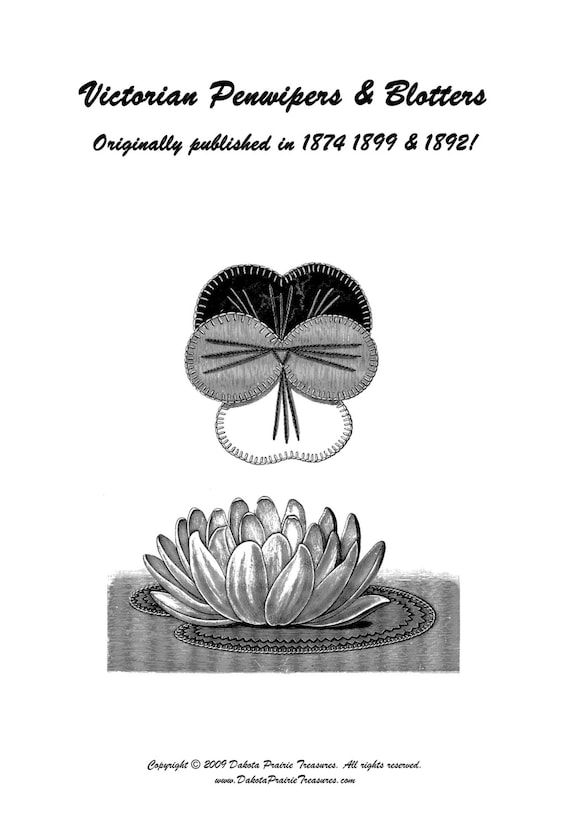This black and white photocopy features the cover of a book titled "Victorian Pen Wipers and Blotters," originally published in 1874, 1899, and 1892, with a copyright notice from 2009 by Dakota Prairie Treasures. The cover art includes an image of ornate, frilly designs that resemble clover leaves in shades of black, grey, and white. Below these designs is a lotus flower delicately resting on a lily pad. The middle section of the image shows what look like two layered cloth items, with the gray one on top appearing somewhat like a figure-eight or a cat's face, complete with stitching that suggests whiskers and a triangular nose. This gray cloth piece has stitching around its edges and is layered over a similarly shaped black object. The entire image, inclusive of detailed stitch patterns and intricate designs, maintains a monochromatic theme of various greyscales.